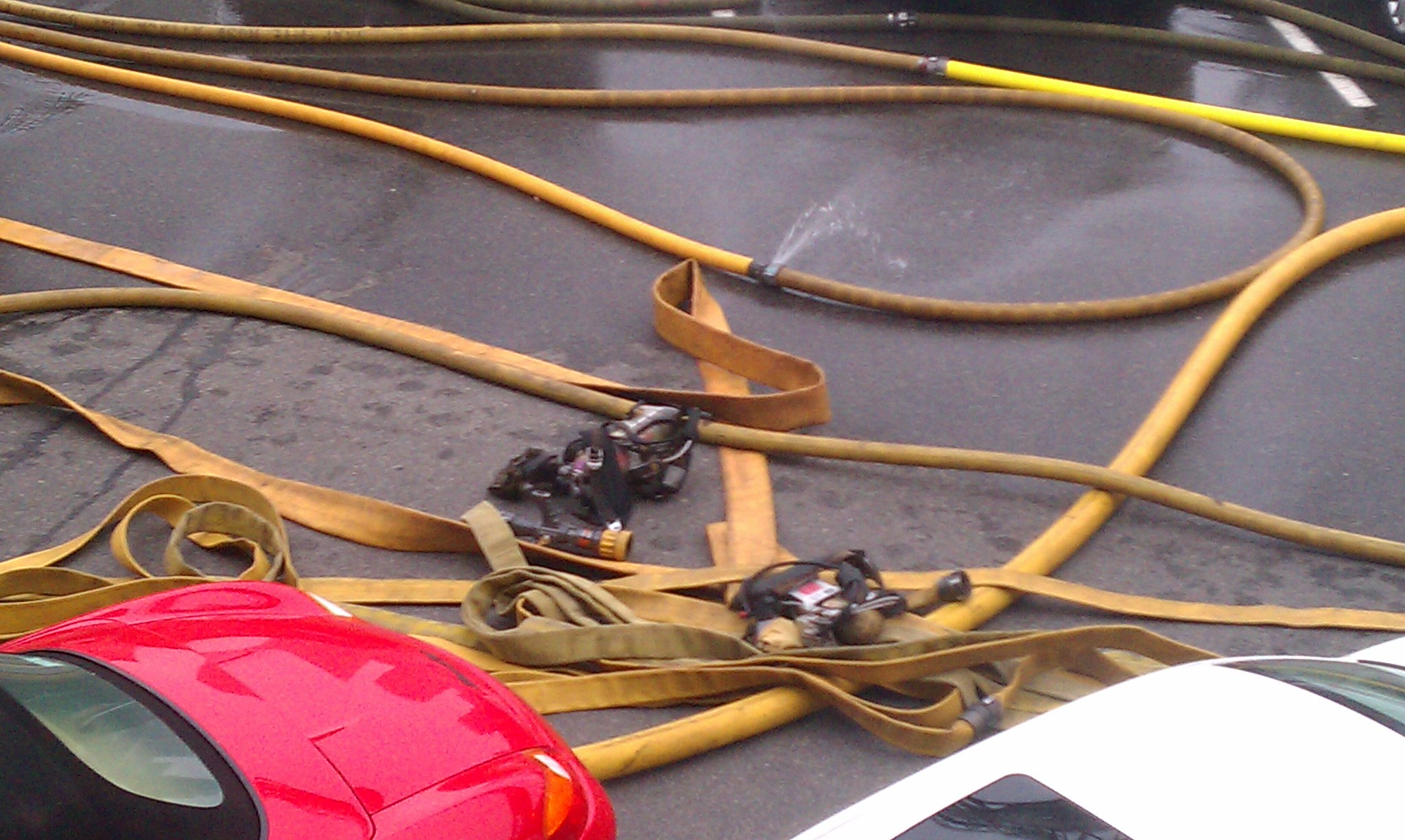This close-up image captures an intricate scene on a black surface, possibly a road or driveway. Yellow hoses, some new and some grungy with age, are entangled together. They are connected to each other, forming a complex network. Notably, at one connection point, water is leaking and spurting into the air, indicating a malfunction. The hoses are associated with a fire truck and show varying states of inflation, suggesting water flow within. Below the hoses, only the sections of two cars are visible: a shiny red sports car with black windows, possibly a convertible, and a white car with a sunroof. The surface appears wet, hinting at recent or ongoing water activity, potentially related to car washing. Additionally, black tape is seen around one of the impaired hose connections, and two black metal objects lie adjacent to the hoses on the partially wet concrete ground.